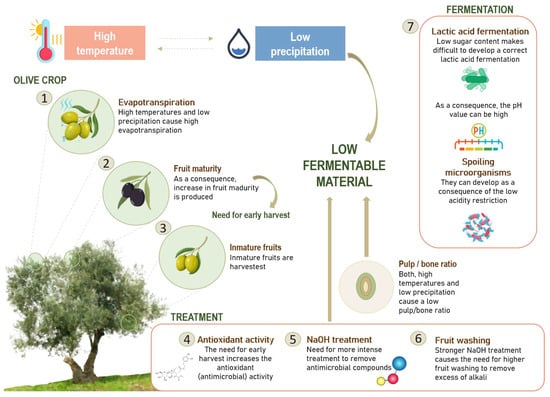An illustrated guide to olive crop processing over a white background. 

In the bottom left corner, a tree on a grassy area is depicted. Above, at the top of the illustration, a red thermometer with a sun icon indicates high temperature, marked by a red block. An arrow points right to an illustration of a water droplet labeled "Low Precipitation." Another arrow loops back from the water droplet to the high-temperature block. Various steps in olive processing are numbered and detailed below these main elements.

Underneath the thermometer, a red label reads "Olive Crop Step 1," accompanied by an illustration of olives on a branch with detailed information about the initial stage. Step 2 shows darker olives, indicating ripeness. Step 3 presents another circle depicting immature olives.

Step 4, located in a block labeled "Treatment," consists of various sub-processes: 
1. Antioxidant activity 
2. NaOH treatment 
3. Fruit washing

Step 7 is housed in another rectangular block under the heading "Fermentation," specifically detailing "Lactic Acid Fermentation," complete with illustrations of the various stages involved. 

An arrow from "Low Precipitation" leads to a label "Low Fermentable Material," directing up and down to the treatment processes. A small circle nearby is annotated with "Pulp to Bone Ratio," completing the detailed overview of the olive crop processing sequence.